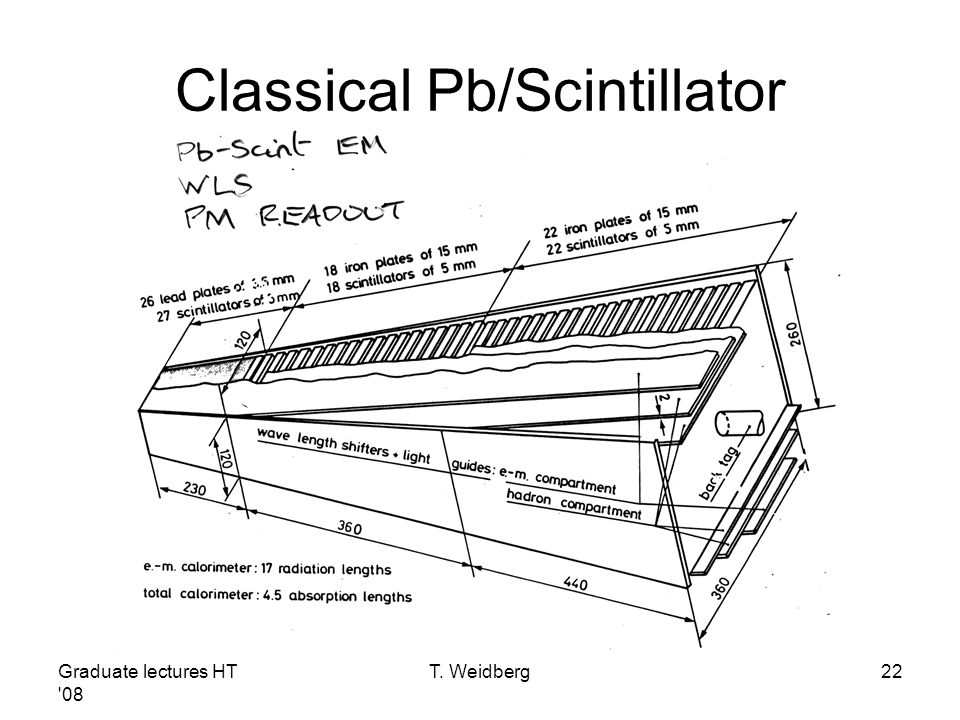This horizontal, black-and-white image features an engineering drawing of a rectangular piece of equipment, likely excerpted from a technical textbook. At the top, the text "classical PB / scintillator" is prominently displayed in black letters, accompanied by handwritten notes that hint at an "afternoon readout." The detailed diagram shows an exploded view of the equipment's interior, with various parts labeled in both English and another language, utilizing two different units of measurement to specify the dimensions of its width and length.

The diagram includes measurements such as "26 lead plates of 35 mm," "25 scintillators of 5 mm," "18 iron plates," and "18 scintillators." It also features distinct ridges and other structural details that are meticulously annotated. Beneath the illustration, text indicates this image is part of "graduate lectures HT 08" by T. Weidberg, specifically found on page 22. The clear presentation of the dimensions and design elements suggests this is a well-detailed educational resource for engineering students.